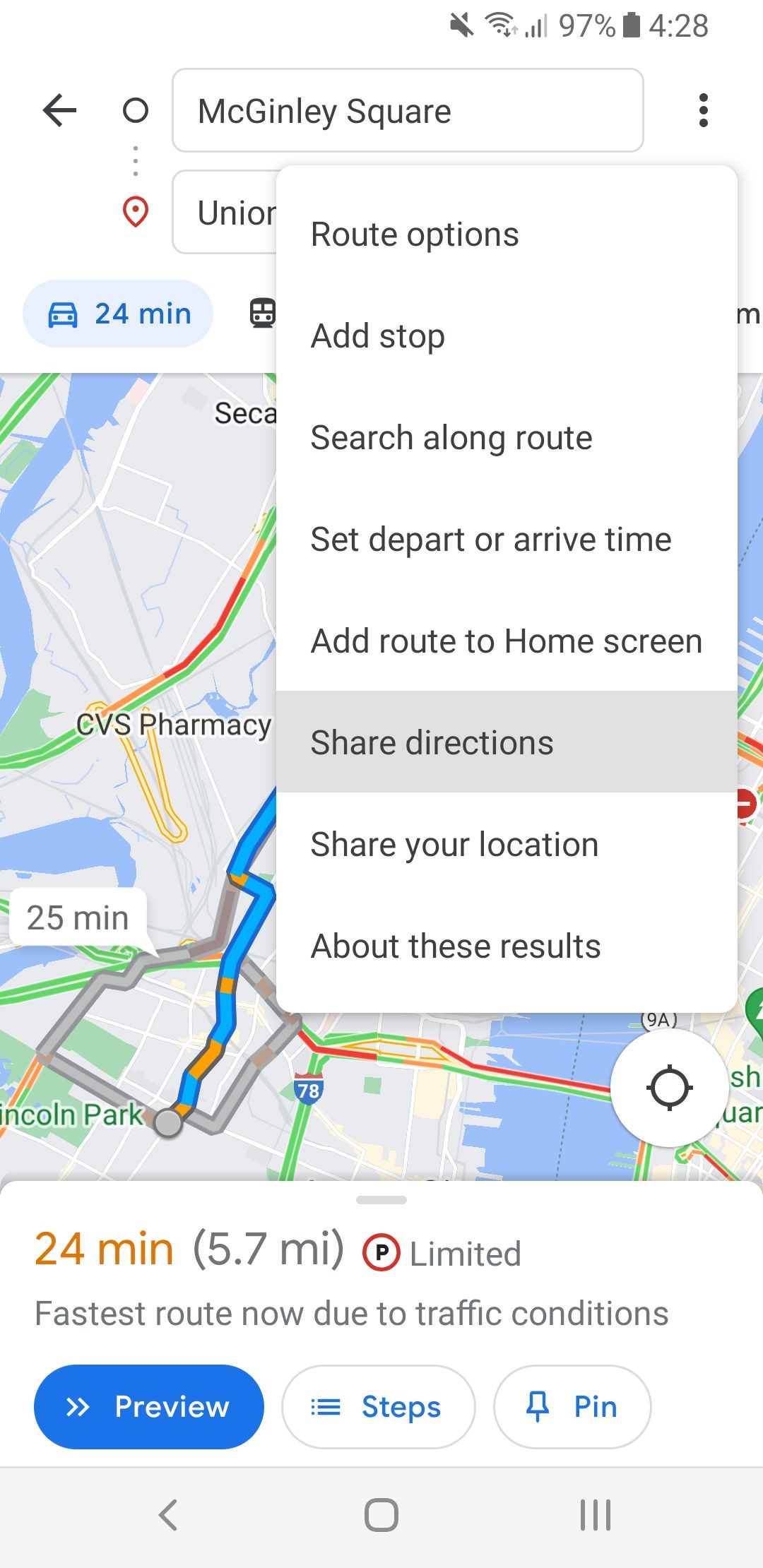The screenshot displays a user interface on a white background with gray icons aligned at the top right. Below, on the left side, there's a black arrow pointing to the left. Adjacent to it is an oval outlined in gray. Further right is a light gray-outlined rectangular box labeled "McGinley Square," accompanied by three vertical ellipses buttons. A dotted line connects the gray-outlined oval to a red circle with a red dot at its center. Near the bottom, another rectangle, similar to the one above, is partially visible with only the letters "UNIO" shown, obscured by a white pop-up box containing a list of options in gray print. 

The list includes:
- Route options 
- Add stop 
- Search along route 
- Set depart or arrive time 
- Add route to home screen 
- Share directions (highlighted with a gray rectangle around it) 
- Share your location 
- About these results

To the left of "Add stop" is a blue oval with a car icon and "24 MIN" in blue. Beneath this, there is a Google map section. Below the map, it shows "24 MIN" in orange, with "(5.7 MI)" in gray. There is a small, bolded black "P" with a red circle around it, followed by the word "limited" in gray. Further below, it notes in gray, "fastest route now due to traffic conditions." At the bottom are three buttons: "Preview" (in blue), "Steps," and "Pin".